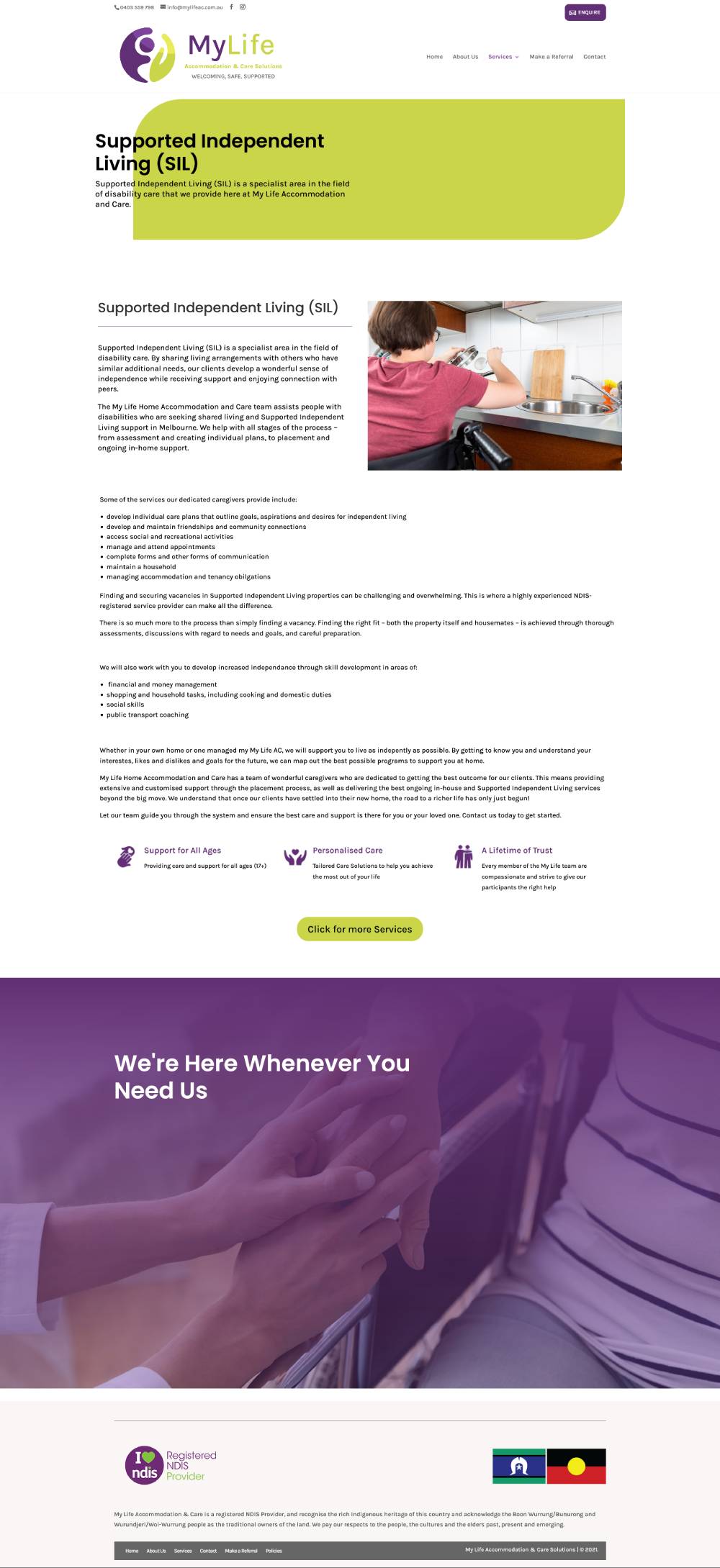This portrait-oriented image consists of two distinct sections that, when combined, form an overall shape approximately two and a half times as tall as it is wide. The image is divided into an upper section and a lower section, each functioning almost as separate pages from an online source.

### Upper Section

The upper section of the image is portrait-oriented and appears akin to a letter or a section from an online news page, though it is more likely from a newsletter. There is no outer border around this section. In the upper left corner, the heading "My Life" is accompanied by a circular logo to its left. This logo is split into two abstract shapes: the left side is purple, and the right side is light green. The text "My" is in purple, and "Life" is in a lighter yellowish-green color, indicating the brand.

Beneath this branding, there are unreadable small texts designed for section selection. Below this, there is a header with a light greenish-yellow curved rectangle, with the top left and bottom right corners curved. Inside this header, the black font reads "Supported Independent Living (SIL)". The phrase "Living in SIL" is on a separate line beneath the header, followed by two and a half lines of smaller text.

Adjacent to this text, on the right side, an image shows a woman in a wheelchair working at a kitchen counter in front of a sink. The image is taken from behind, offering a view of her back. The rest of the section comprises a newsletter-like article titled "Supported Independent Living (SIL)". This article contains several paragraphs of informative text and five to six bullet points in the middle, providing detailed insights on the topic.

### Lower Section

The lower section of the image is landscape-oriented and presents a large picture occupying the top two-thirds of its space. The background is a purplish-lavender hue, and the image features a close-up of an individual in a wheelchair. The visible portions include the right armrest of the wheelchair and the person's torso, with their right arm resting on the armrest. Notably, two additional hands appear from the lower left, connecting with the wheelchair user's hand, signifying assistance.

Beneath the image, a gray rectangular section includes text and colorful images, including flags. These elements likely provide additional context or information relevant to the overall content presented in the image.

Overall, this composite image offers detailed information about Supported Independent Living (SIL) and visually portrays assistance provided to individuals in wheelchairs, combining textual and visual elements seamlessly.